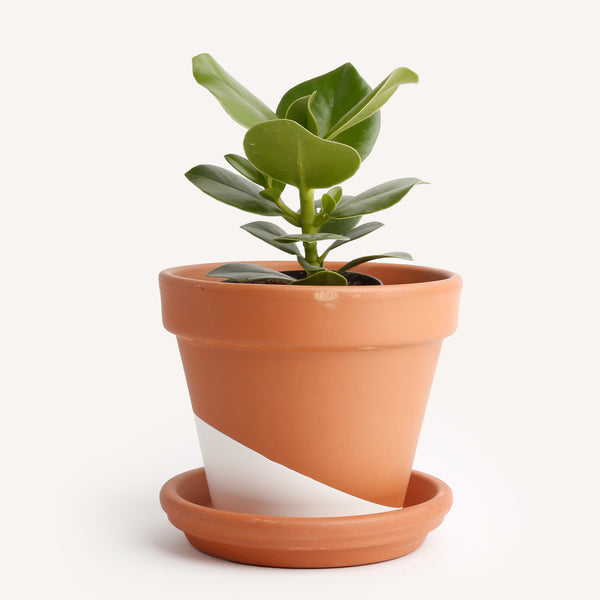This photograph showcases a small, sturdy, tropical plant with wide, pointed, green leaves, standing about 4 inches tall. It is potted in a distinct, orange terracotta pot with a white diagonal stripe on the lower left corner, sitting atop a matching orange plate. The thick-stemmed plant, which appears to resemble an ivy variety, is set against a light off-white background. The pot has a unique design, further highlighted by the stripe, and includes a water-catching dish beneath it. The overall scene is clean and simple, focusing entirely on the charmingly modest potted plant.